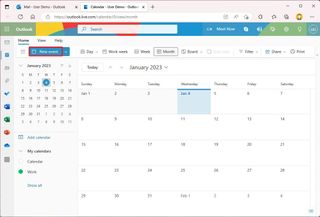The image features a screenshot of a Microsoft Office calendar. On the left-hand side, there's a smaller calendar display with today’s date circled and highlighted in blue. The main section showcases a larger calendar for January 2023. This calendar is labeled with color-coded entries in green, yellow, red, and blue, although no specific events are described within the image. The date "January 3rd" is distinctly highlighted in blue. Above the calendar, Microsoft Office icons are clearly visible in full color, indicating various available functionalities. Despite attempts to enlarge the image for a clearer view, the text becomes blurry, keeping the detailed content indiscernible. The overall color scheme includes a gray background area, adding subtle contrast to the vividly colored icons and calendar entries.